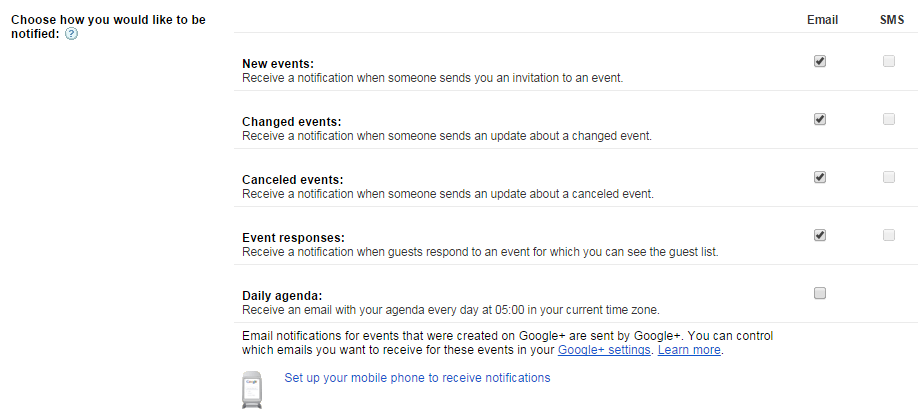The image showcases a white canvas displaying various options for notification preferences related to events, arranged in a structured, top-to-bottom format. Here is a detailed description of the text content and options available:

1. **Notification Preferences:**
   - **News Event:** 
     - Description: Receive a notification when someone sends you an invitation to an event.
     - Options: Email (checked), SMS.
   - **Changed Events:**
     - Description: Receive a notification when someone sends an update about a change in an event.
     - Options: Email (checked), SMS.
   - **Canceled Events:**
     - Description: Receive a notification when someone sends an update about a canceled event.
     - Options: Email (checked), SMS.
   - **Event Responses:**
     - Description: Receive a notification when guests respond to an event for which you can see the guest list.
     - Options: Email (checked), SMS.
   - **Daily Agenda:**
     - Description: Receive an email with your daily agenda at 05:00 AM in your current time zone.
     - Options: Email (unchecked).

2. **Additional Information:**
   - Note: "Email notifications for events created on Google Plus are sent by Google Plus. You can control which emails you want to receive for these events in your Google Plus [settings](hyperlinked), and also [learn more](hyperlinked)."

3. **Illustration and Instructions:**
   - At the bottom, there is an illustration of a phone accompanied by the text: "Set up your mobile phone to receive notifications."

This detailed caption highlights the hierarchical structure of the notification options and provides clear instructions and additional information, ensuring comprehensive understanding for the reader.